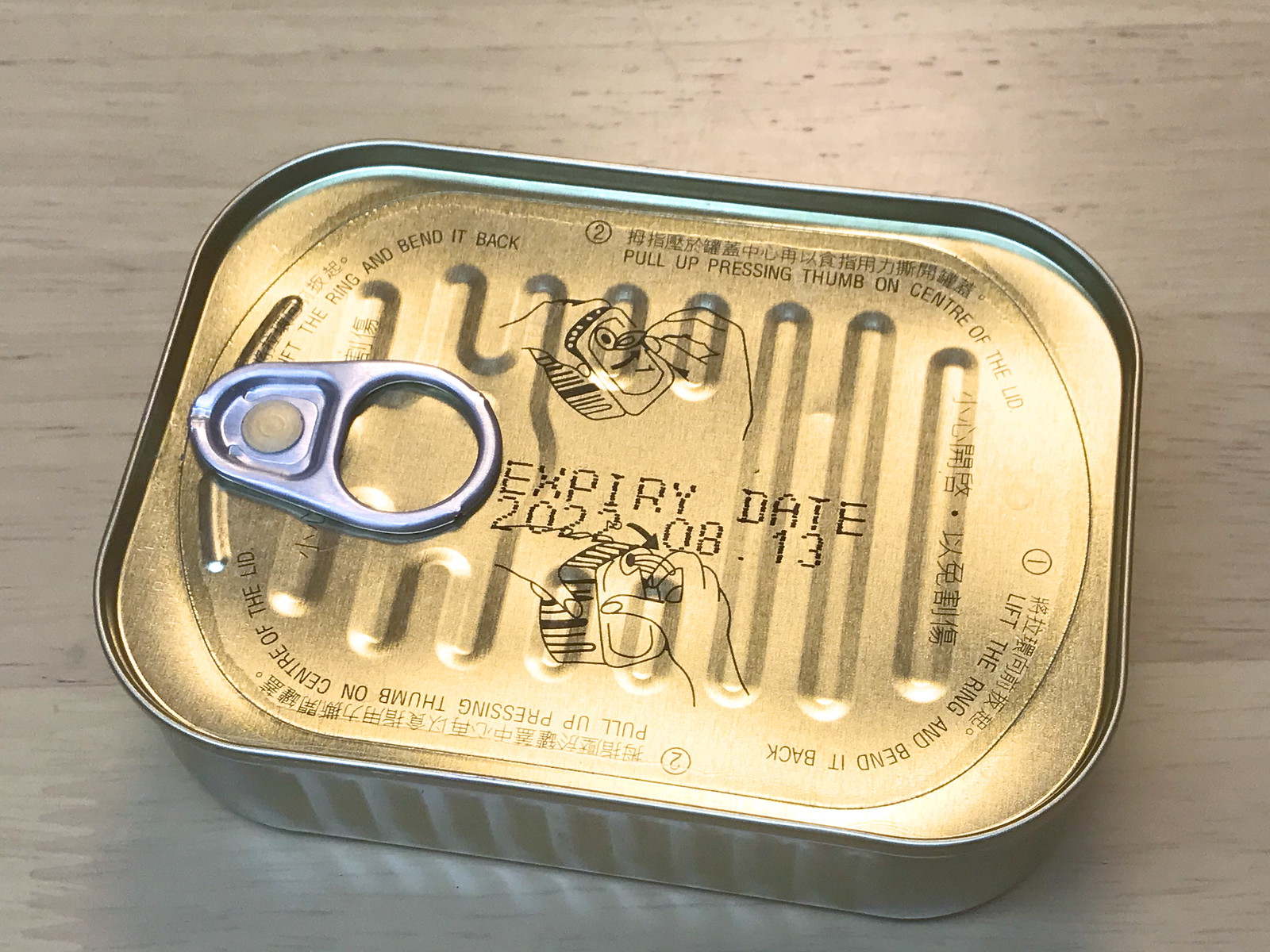The image depicts a rectangular sardine can with rounded edges, positioned in the lower center of a light brown wooden surface that features subtle horizontal black markings. The can itself has a coppery-gold tint and features a pull-back aluminum tab on the top, designed for easy opening without a can opener. Detailed instructions, both in English and what appears to be Japanese kanji, illustrate how to lift the ring and bend it back to open the can with a visual aid showing a hand performing the action. Prominently displayed on the top is the expiration date, reading 2022-08-13. The entire scene captures the unopened can, emphasizing the convenience of its design and the clear, multilingual directions for use.